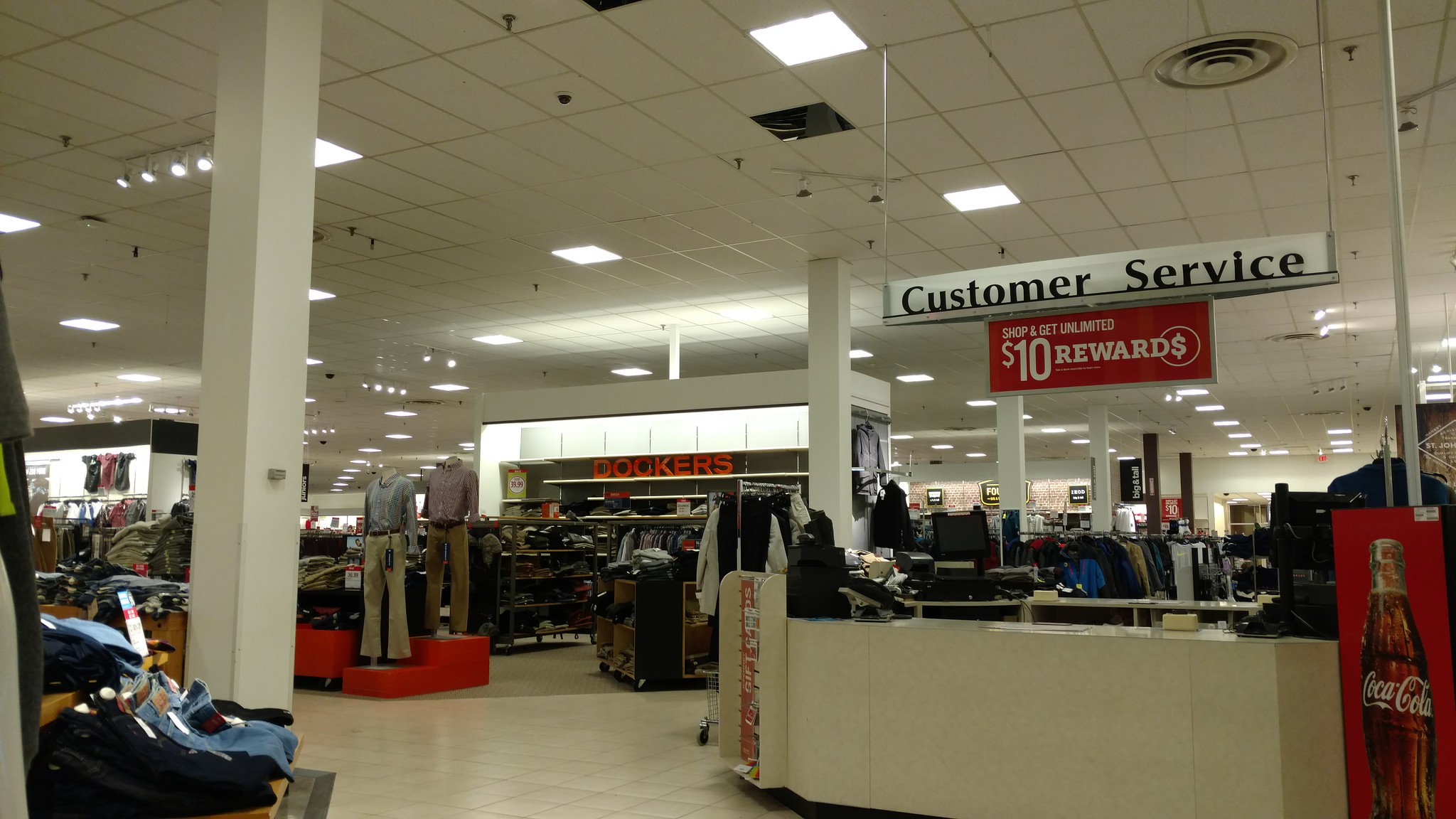The image depicts the interior of an unidentified clothing store. To the right, a ceiling-mounted sign prominently displays "Customer Service," guiding shoppers to a counter below where they can check out their clothing and other items. Beneath this sign, another message encourages customers to "Shop and get unlimited $10 rewards." The store is filled with a variety of clothing items; to the left, there is a section showcasing jeans, and nearby, there's an area dedicated to men's apparel. The overall scene is bustling with a diverse assortment of clothes arranged neatly, creating an inviting shopping environment.